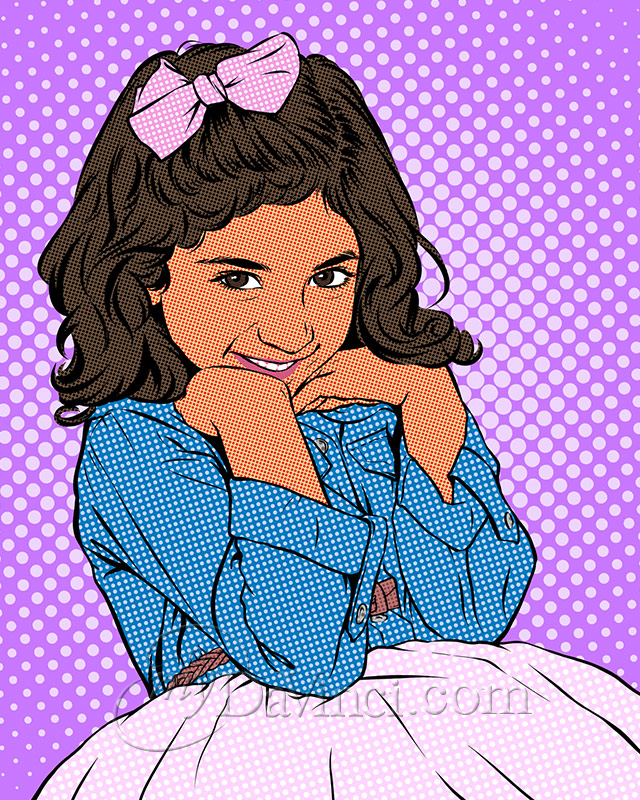The image is a comic book-style drawing with pixelated coloring featuring a young girl who appears to be six or seven years old. She has a slightly darker complexion, possibly Latina, with dark brown, wavy shoulder-length hair adorned with a pink bow. Her large brown eyes and coy smile add to her happy appearance. She is dressed in a blue long-sleeve button-down shirt, cinched at the waist with a thin brown leather belt, and a puffy pink skirt that is visible just past her waist. Both of her hands are positioned under her chin, elbows bent, and she is smirking at the viewer. The background is a purple field with hundreds of white dots scattered across it, adding to the whimsical feel of the illustration. There is a watermark that says "DaVinci.com" on the image.